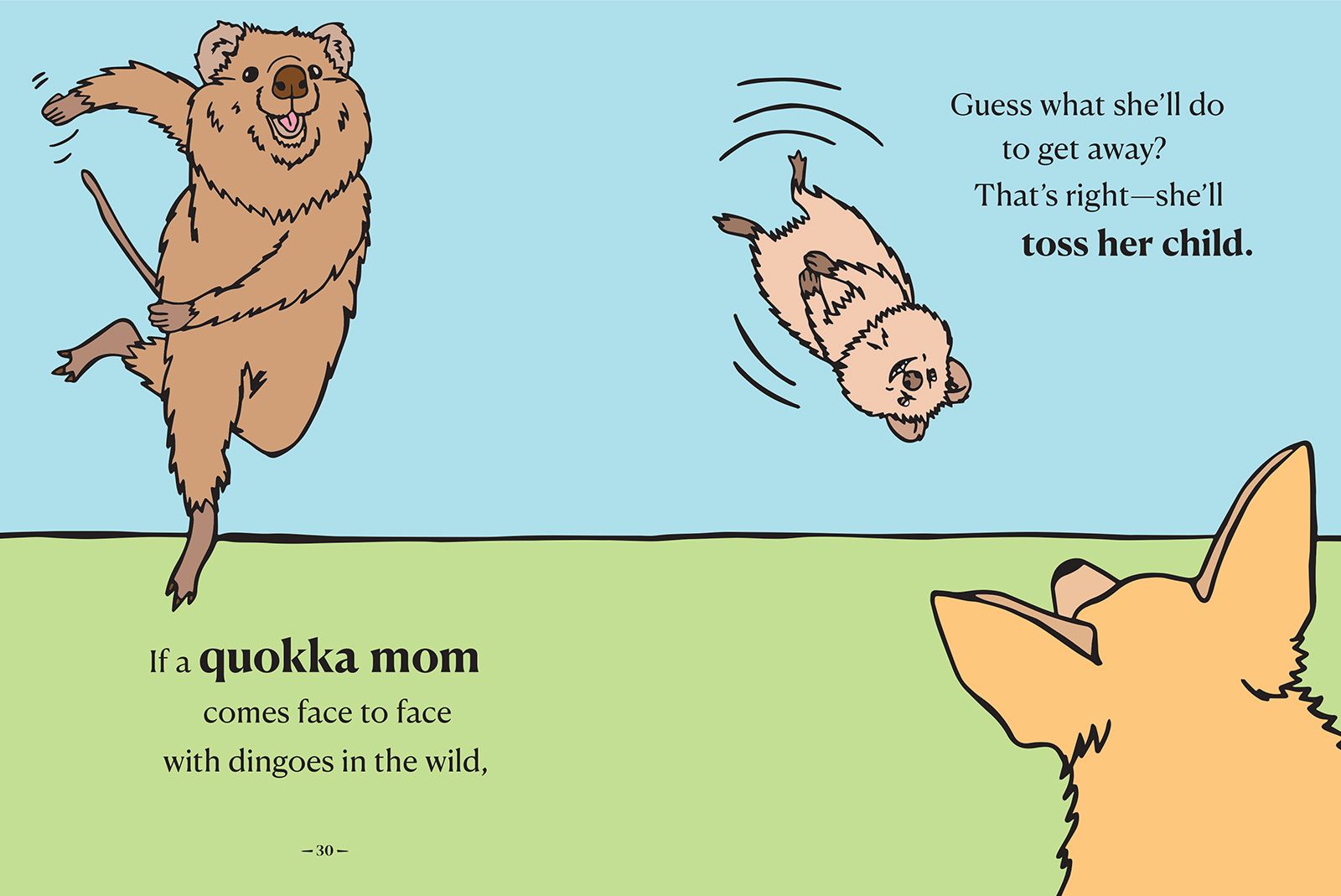The image is a colorful cartoon illustration in a wide vertical rectangular format. The background features a light blue sky occupying the top two-thirds of the image, while the bottom third is light green, representing grass, with a black horizontal line dividing the sky from the grass. On the left side of the image, a bear-like creature stands upright, engaging in a throwing motion with its left leg bent back and arms swinging, giving a human-like posture. This creature has darker beige fur and a joyful expression on its face.

Towards the upper right, a smaller, light beige bear is depicted mid-air, upside down, and diagonal with lines of motion, and a smile on its face indicating its unaware state. The smaller bear appears to be thrown towards the lower right corner where a dingo, a dog-like creature, stands looking up at the flying bear with its mouth open in anticipation and ears pointed upwards.

Text accompanies the image, formatted with specific phrases in strategic locations. Below the larger bear on the left, it reads, "If a quokka mom comes face-to-face with dingoes in the wild," while in the upper right-hand corner next to the flying infant bear, the text continues, "Guess what she'll do to get away? That's right, she'll toss her child." Notably, "toss her child" is emphasized in bold type.

The playful yet dark nature of the illustration is encapsulated by the dynamic depiction of the animals and the illustrative style, rendering a vivid scene set against the simple, contrasting backdrop of sky and grass.